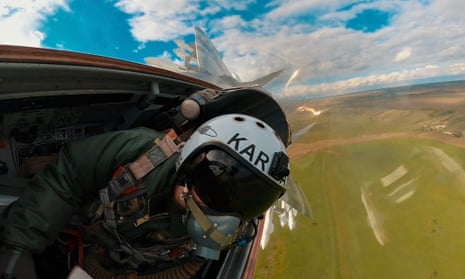The image depicts a pilot in a fighter jet, captured from a pilot cam perspective looking directly at them. The pilot, whose gender is assumed male, wears a dark green jumpsuit with a strap over one shoulder. He is adorned with a white helmet bearing the letters "K-A-R" in black text and a black visor covering his face. Tannish skin is faintly visible behind a green oxygen mask secured with green straps. The jet is knifing sideways with two tail fins, suggesting its high speed and agile maneuvers. In the background, a partly cloudy blue sky extends above a patchwork of green and brown earthy fields below, indicating a relatively low altitude with no visible buildings or structures.